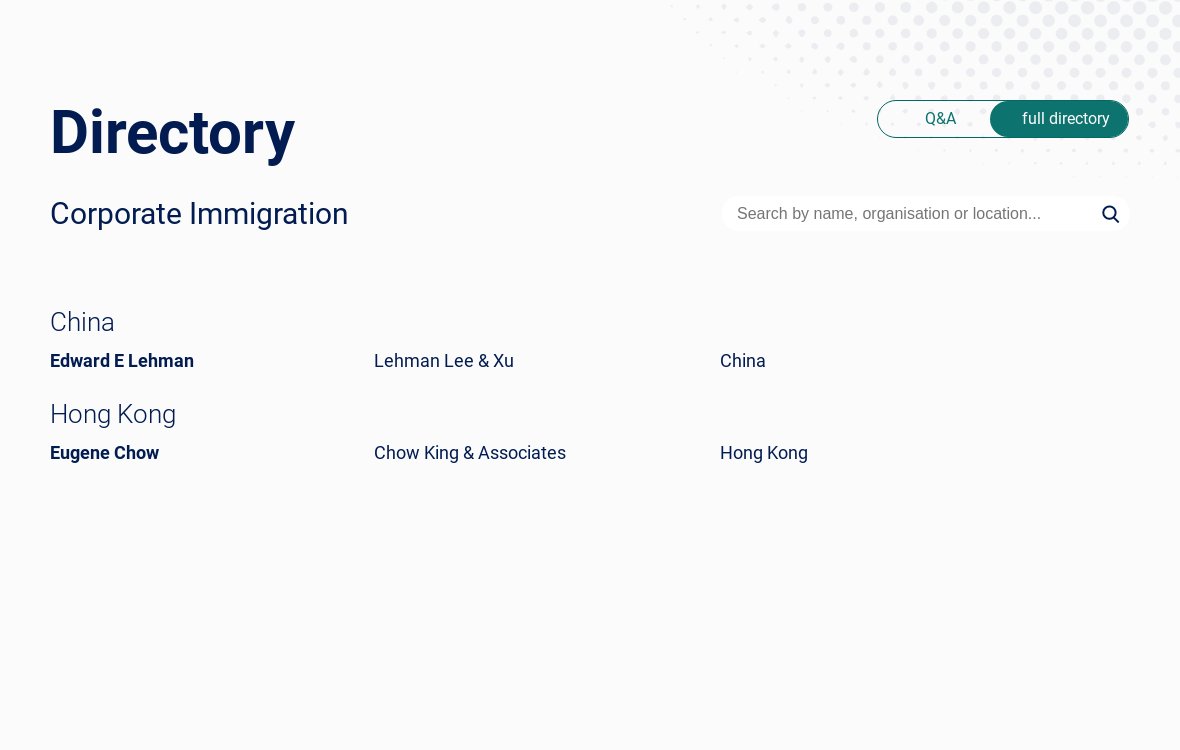Certainly! Here's a refined and detailed caption:

---

In this image, we see a screenshot displayed on a clean white background. The upper right corner features a graphic design composed of varying sizes of grey dots arranged in rows, diminishing in size as they extend to the left. Directly below this graphic is a bi-colored button: the left side is white with the text "Q&A," while the right side is green bearing the text "Full Directory."

In the upper left corner of the screenshot, large bold text reads "Directory." Directly beneath this title, the subheading "Corporate Immigration" is displayed. Adjacent to this, on the right side, there is a search bar with a placeholder prompt in light grey text that says, "Search by name, organization, or location," accompanied by a magnifying glass icon.

Below this search bar, the directory entries are listed. The first entry on the left is for "China," followed by the name "Edward E. Lehman." Correspondingly on the right, the associated firm "Lehman, Lee, and Xu" is indicated, with the location specified again as "China."

Further down on the left, a second entry is listed: "Hong Kong" and the name "Eugene Chow." This is followed by the firm name "Chow King and Associates," with the location reiterated as "Hong Kong."

---

This refined caption provides a thorough description of all the visual and textual elements present in the image, clearly organizing the information for better understanding.